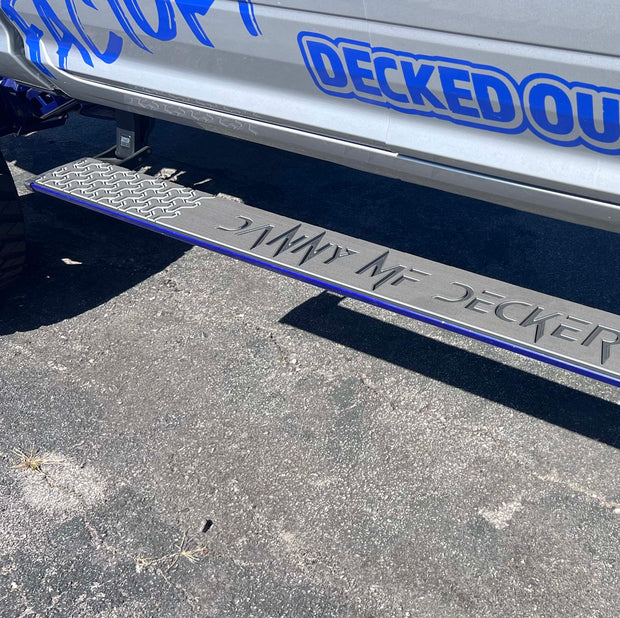The image depicts a rugged, silver pickup truck with a prominent, metal side step designed to assist in entering the vehicle. The truck is adorned with eye-catching blue graffiti-style text that reads "DECKED OUT," with blue outlines emphasizing the phrase on the silver-gray metallic surface. On the stainless steel side step, which features a textured, traction-enhancing surface resembling sandpaper, there are squiggly lines for grip and the words "DANNY M.F. DECKER" etched, with the lightning bolt-style 'N's adding a distinctive touch. The lower half of the image shows cracked, black asphalt with patches of lighter gray and dead weeds protruding from some of the crevices. The step itself is aligned diagonally across the width of the image, further enhancing the detailed representation of both the truck and its step on the worn pavement.